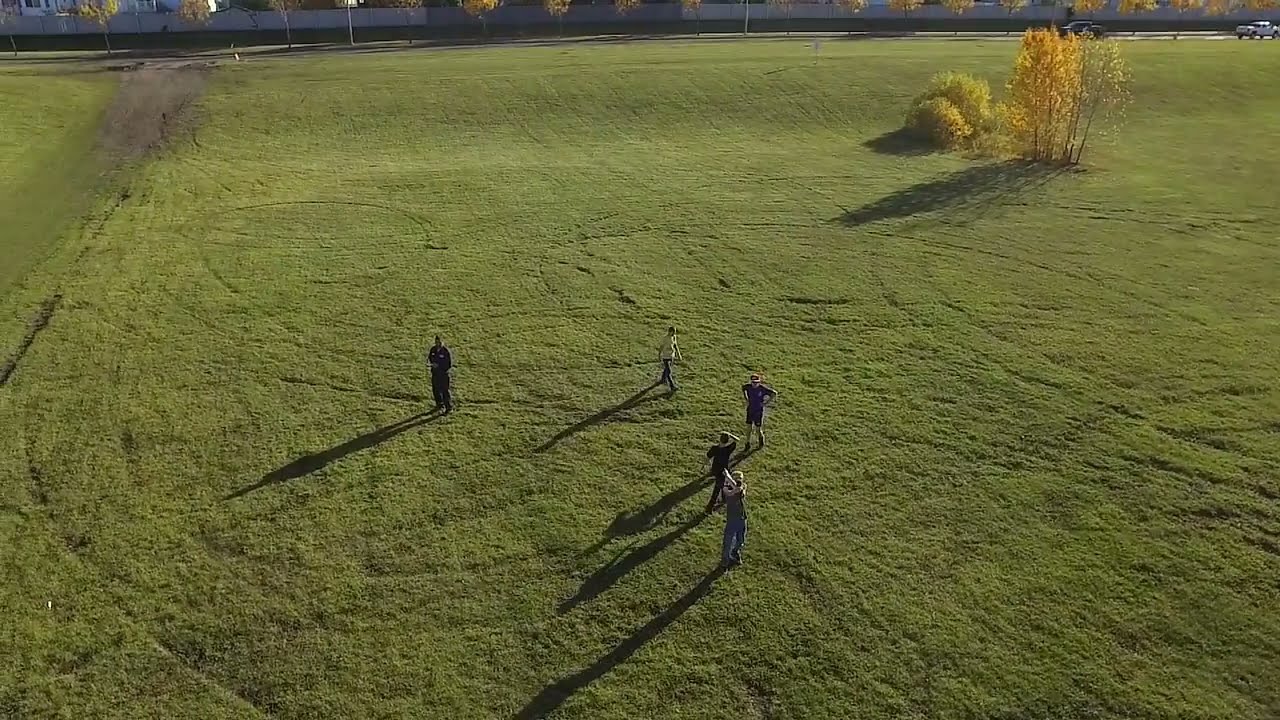This image captures an aerial view of a large grassy field where five young individuals are dispersed across the area. They are mostly clad in dark clothing, with one individual in the center wearing a yellow t-shirt. The person in the bottom center holds something over their shoulder, while another stands with their hands on their waist, and one more in the background touches his head. Their shadows stretch towards the bottom left, indicating sunlight coming from the top right corner of the image.

In the top right, a mix of green, yellow, and brown trees, with some bushes, create a natural border for the field. On the top left, there is a dirt pull-in area and possibly a residential setting in the background. A long dirt road runs parallel to the field, where a white pickup truck and a black pickup truck drive in the top corners of the image. The field itself shows various vehicle markings, curves, and circular patterns imprinted on the grass, hinting at previous activities, likely from vehicles such as dirt bikes or four-wheelers. Overall, the scene suggests a rural environment with a touch of human presence mingling with nature.